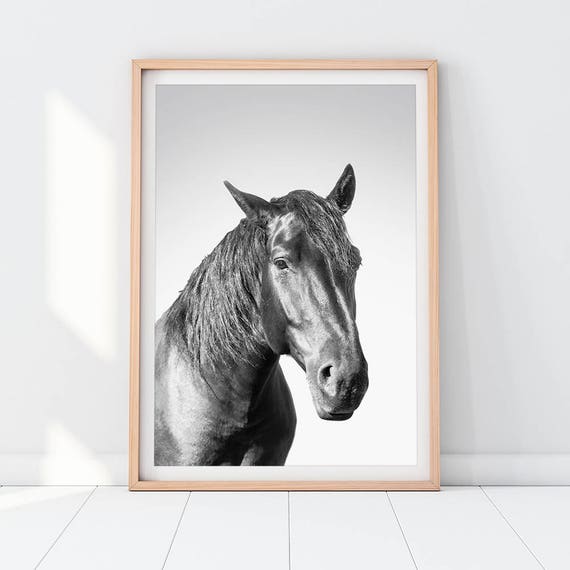This is a black and white portrait of a horse, beautifully captured and displayed within a light natural wood frame. The photograph reveals a close-up of the horse's face, showcasing its expressive eyes and black mane, which convey a sense of sadness and loneliness. The tall pointy ears add to its dignified presence. The image appears to be propped against a white wall, resting on a wooden surface that resembles a shelf or floor. Sunlight streaming in from a nearby window creates a warm reflection on the wall and across the lower part of the photograph, enhancing the serene yet melancholic mood of the scene. The picture's intricate details are enveloped by a white border, adding a subtle elegance to its presentation.